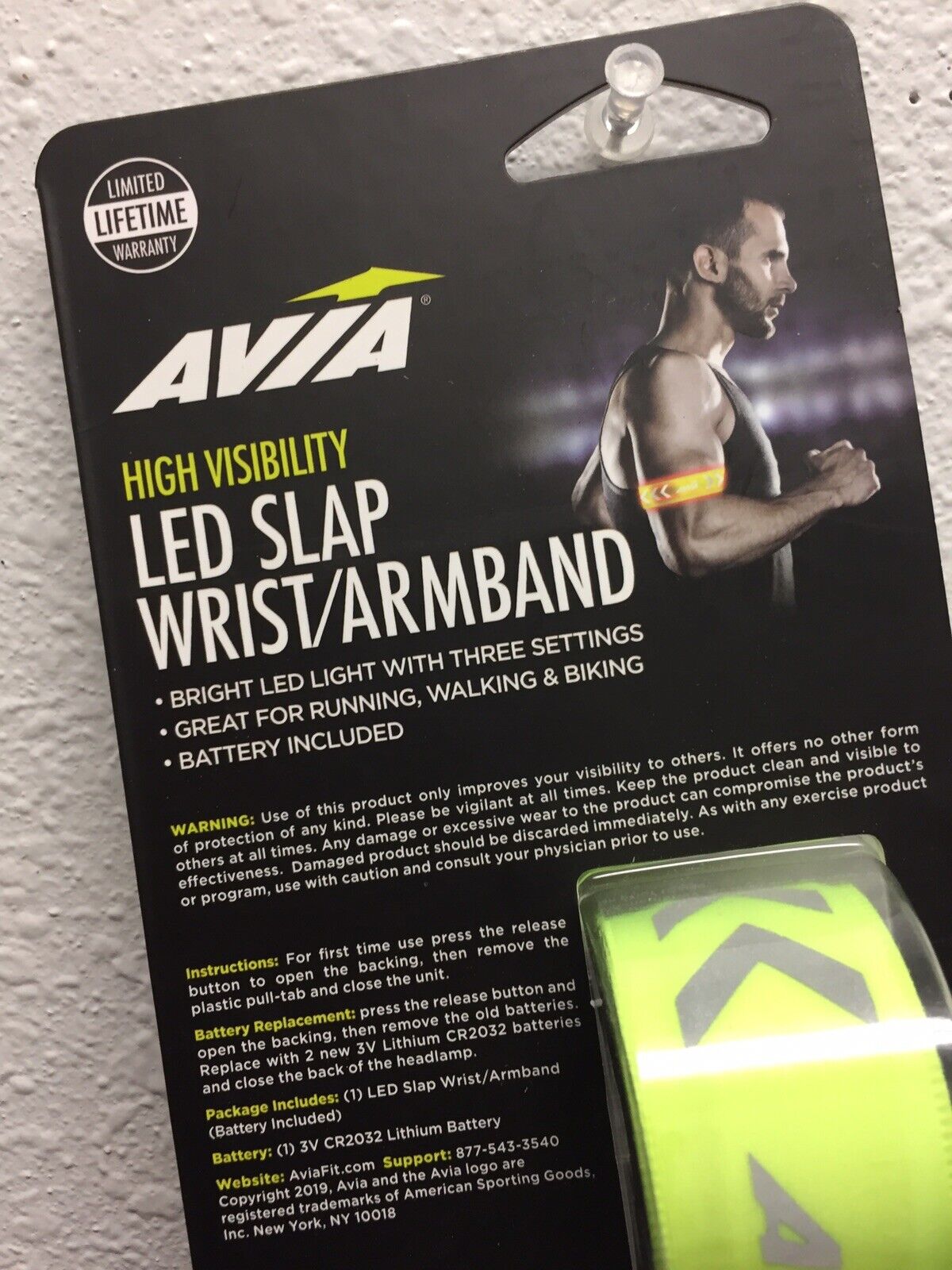The image showcases the product packaging for a high-visibility LED slap wrist/armband by Avia. The packaging, which is a black cardboard placard adorned with white and yellow lettering, features the Avia brand prominently at the top. Encased in a transparent plastic blister pack is the fluorescent yellow armband, coiled neatly for display. In the upper right corner, there's a photograph of a muscular man running, with the armband securely fastened around his upper right arm. This man is depicted from the chest up, with his arm bent at a right angle and his fist near his chest. The packaging highlights key product features: a bright LED light with three settings, ideal for running, walking, and biking, with the battery included. A circle in the upper left corner of the packaging mentions a Lifetime Limited Warranty. Below the product name, bullet points emphasize these features. A warning section, with "Warning" in yellow text, advises that the product only improves visibility and offers no additional protection. Instructions for first-time use and battery replacement are also detailed, alongside cautions about product maintenance and consultation with a physician before usage. Packaging details include an included CR2032 lithium battery, Avia's support contact information, and trademark details.